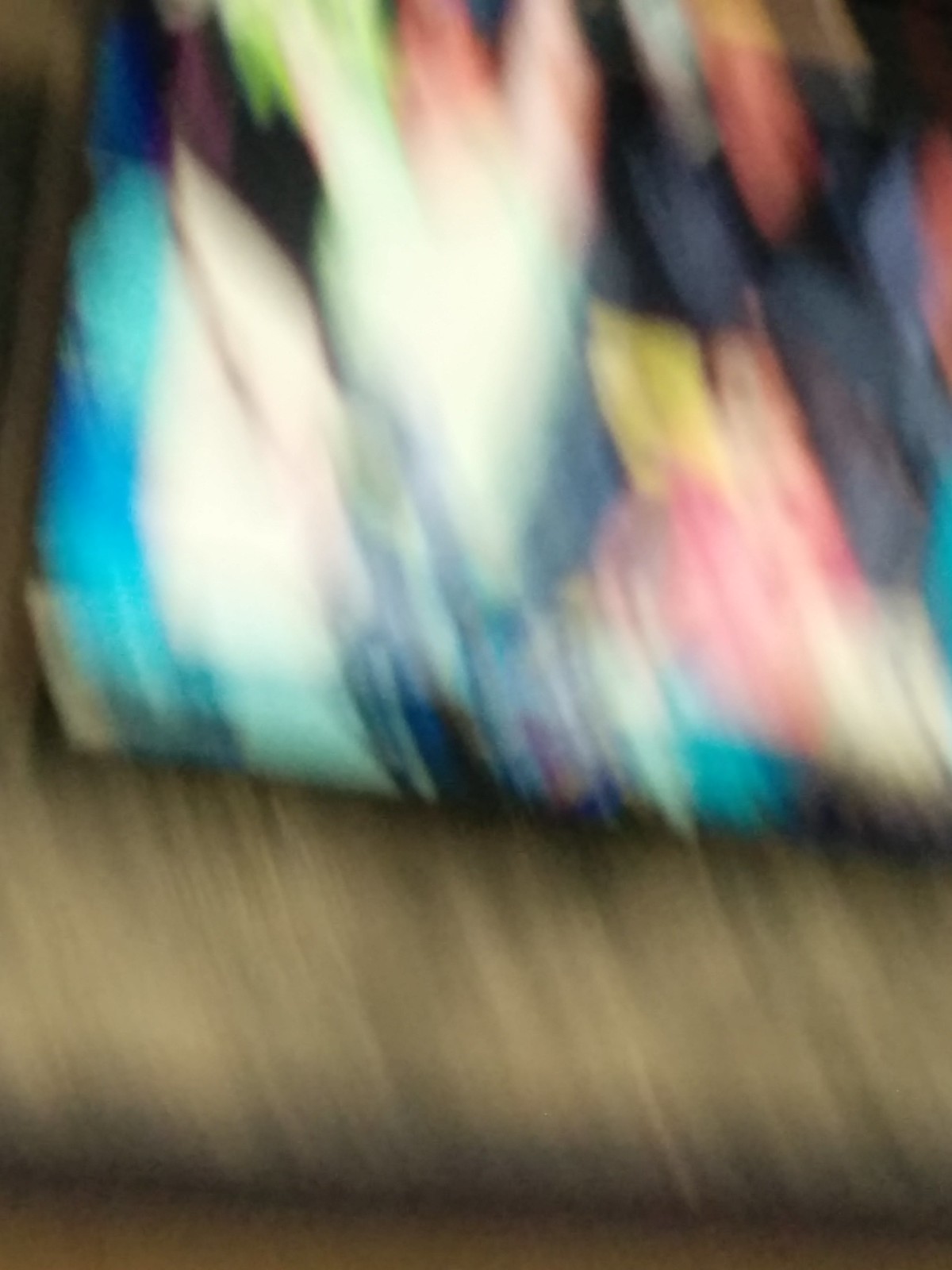A color photograph captures a scene that features a blurred view. Dominating the bottom half of the image is a straight, brown object, likely a fallen tree log, which gradually transitions from a darker brown at its base to a lighter tone above. Situated behind this log are two individuals. One, donning a white shirt, has their hands raised above their head, their face visible despite the overall blur. Beside them, another person wears a blue jacket and seems to be accompanied by several packages. In the background, a mixture of green hues and other colors suggests a distant, possibly natural setting.